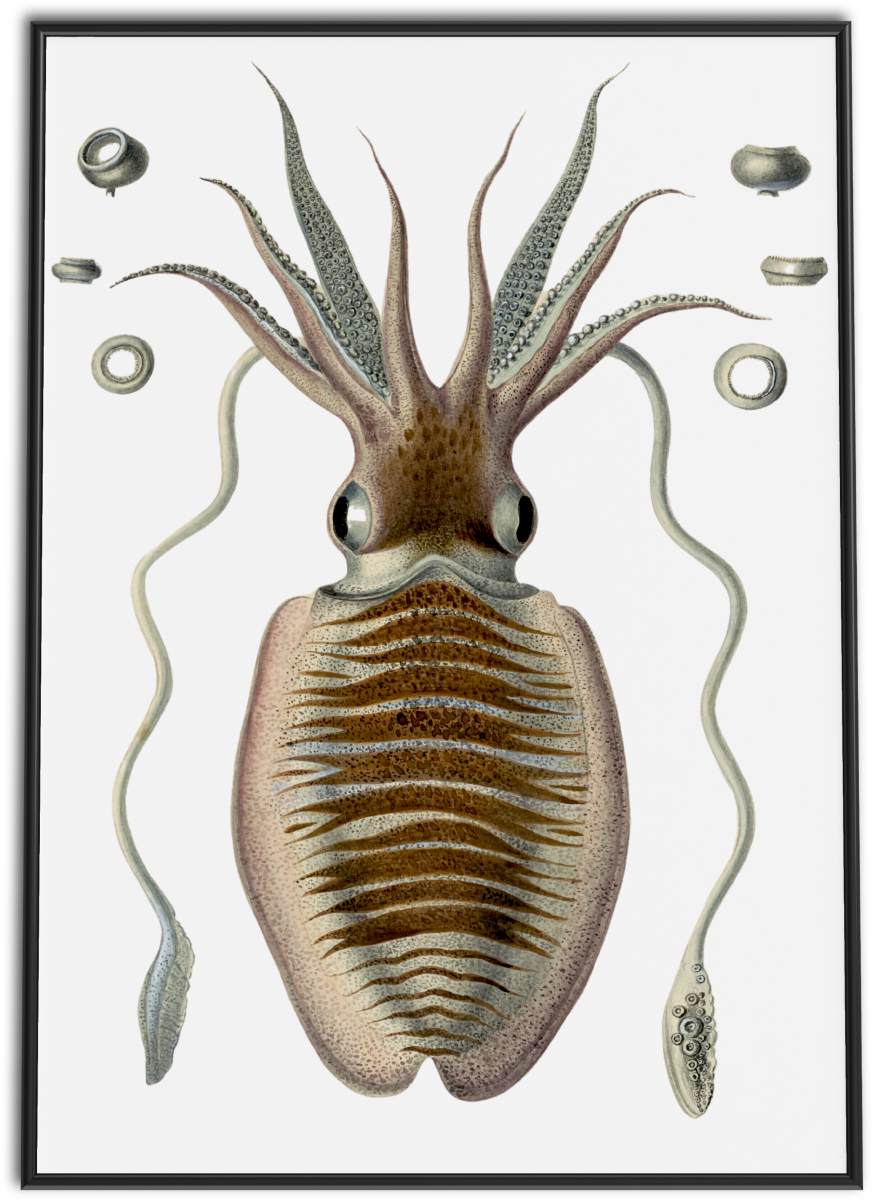The detailed digital illustration, framed with a thin black border, features a fantastical or possibly extinct sea creature, reminiscent of a squid or octopus. The creature, depicted in beige and tan hues with dark brown stripes running along its bulbous, elongated head, stares out with two eyes located near its center. Above the eyes, a series of tentacles extend outward, comprising shorter tentacles and two notably long ones that taper down toward the bottom of the image. Interspersed around the creature are metallic rings, positioned on either side, seemingly suspended in the white backdrop. The illustration's minimalist use of color emphasizes the intricate detailing of the creature's body and tentacles, conveying an otherworldly or prehistoric essence.